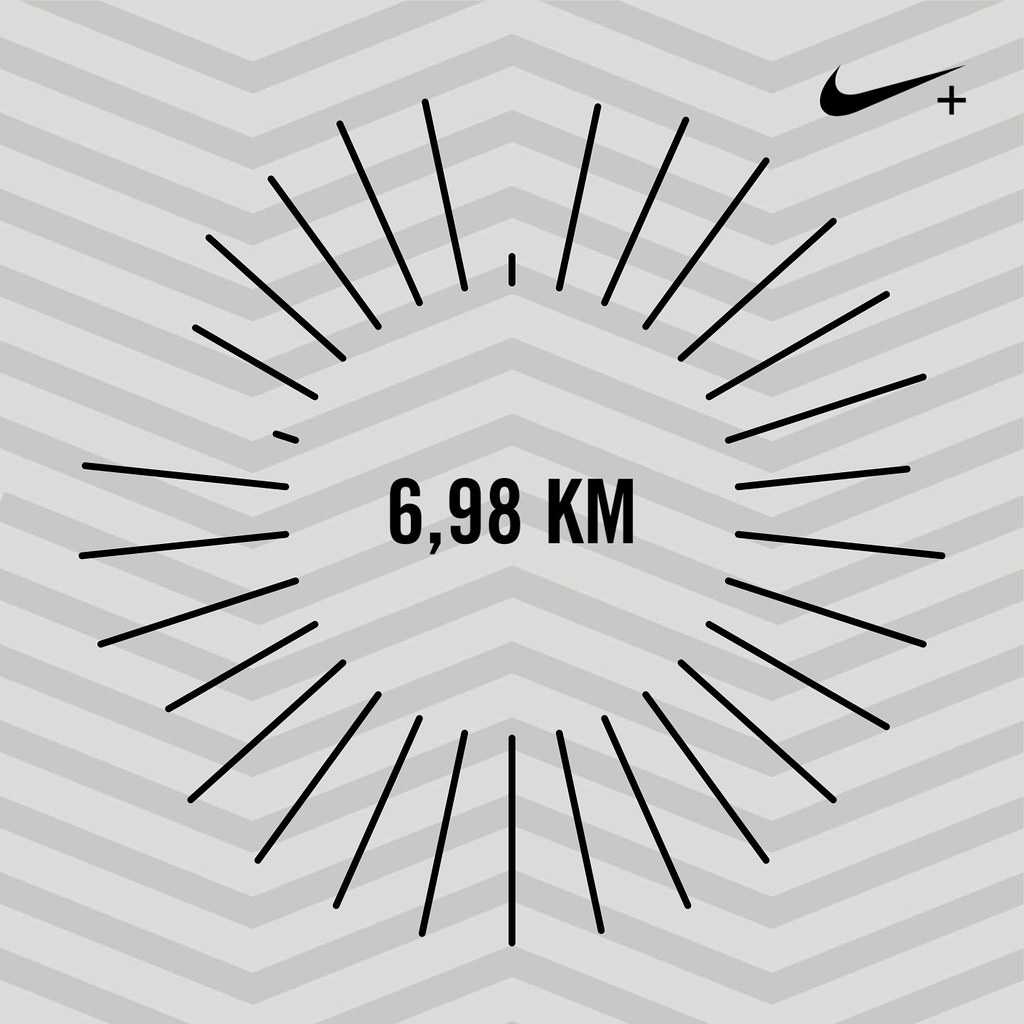The advertisement image features a minimalist design with a light gray background adorned with a darker gray chevron pattern, creating a dynamic texture with sharp points facing alternating directions. At the top right corner, the iconic black Nike logo is displayed, accompanied by a small plus sign situated at the top of the swoosh. Dominating the center of the image is the bold, black text "6,98 KM," indicative of kilometers traveled, which is encircled by radiating black lines resembling sun rays or a burst pattern. These lines vary in length, with two of them, located at the 12 o'clock and between the 10 o'clock and 11 o'clock positions, being noticeably shorter, along with five slightly shorter lines in between. The overall design is clean and striking, emphasizing the key elements through contrast and repetition.